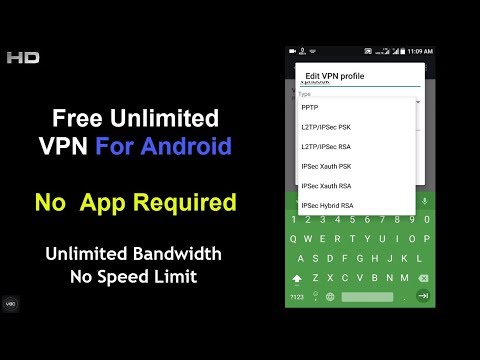Here is the enhanced and detailed caption based on your given description:

---

The image features a black background with various textual elements and an illustration of a cell phone interface. In the upper left corner, the text "HD" is prominently displayed. Below this, the text "Free Unlimited VPN" appears in white, followed by "For Android" in blue. Underneath this line, there's a yellow text stating "No app required". Below that, in white text again, it reads "Unlimited bandwidth, no speed limit." 

There is also a small button outlined in gray that appears to have text, which is difficult to decipher but might say "Login". 

The main part of the image shows an outline of a cell phone, with a pop-up screen overlaying the top portion. The pop-up is an "Edit VPN Profile" window with a green border. It lists various VPN types, including:
1. PPTP
2. L2TP/IPSec PSK
3. L2TP/IPSec RSA
4. IPSec XAUTH PSK
5. IPSec XAUTH RSA
6. IPSec Hybrid RSA

Below this, there appears to be another overlay, showing the word "Type" with a small arrow icon next to it, and an on-screen keyboard with green background and white letters and numbers.

At the very top of the phone display, the time reads "11:09" alongside the battery indicator and signal bars, indicating the interface is portraying a typical cell phone status bar.